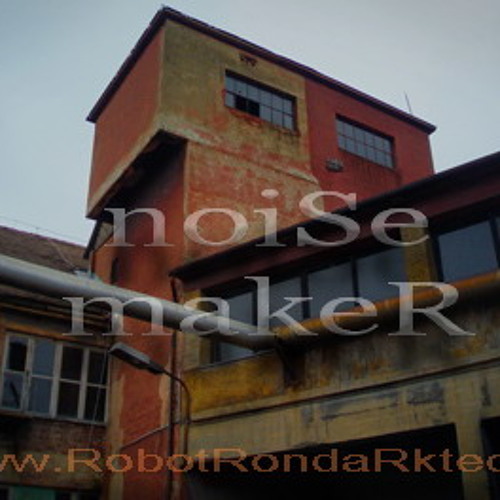This image depicts a dilapidated, industrial-style building captured from the ground looking upward, showcasing its worn and rundown state. The structure appears to have two levels, resembling an old factory with rust and faded paint, primarily in brick red but also featuring patches of dirty yellow, black, and gray. A large, dirty yellow section of the wall has opaque windows set into it, some of which are broken. At the bottom of the image, light-colored text reads "W.ROBOT.RONDA.R.KET," although parts are cut off at the edges. Superimposed over the center of the photograph is the word "NOISEMAKER" in a light, translucent white font, with the S in NOISE and the R in MAKER capitalized. A rusted pipe runs along the wall and juts out to the left, passing by a broken streetlight positioned slightly forward in the foreground. The overall setting suggests a neglected and decayed area, emphasizing the building's long-term exposure to the elements and lack of maintenance.